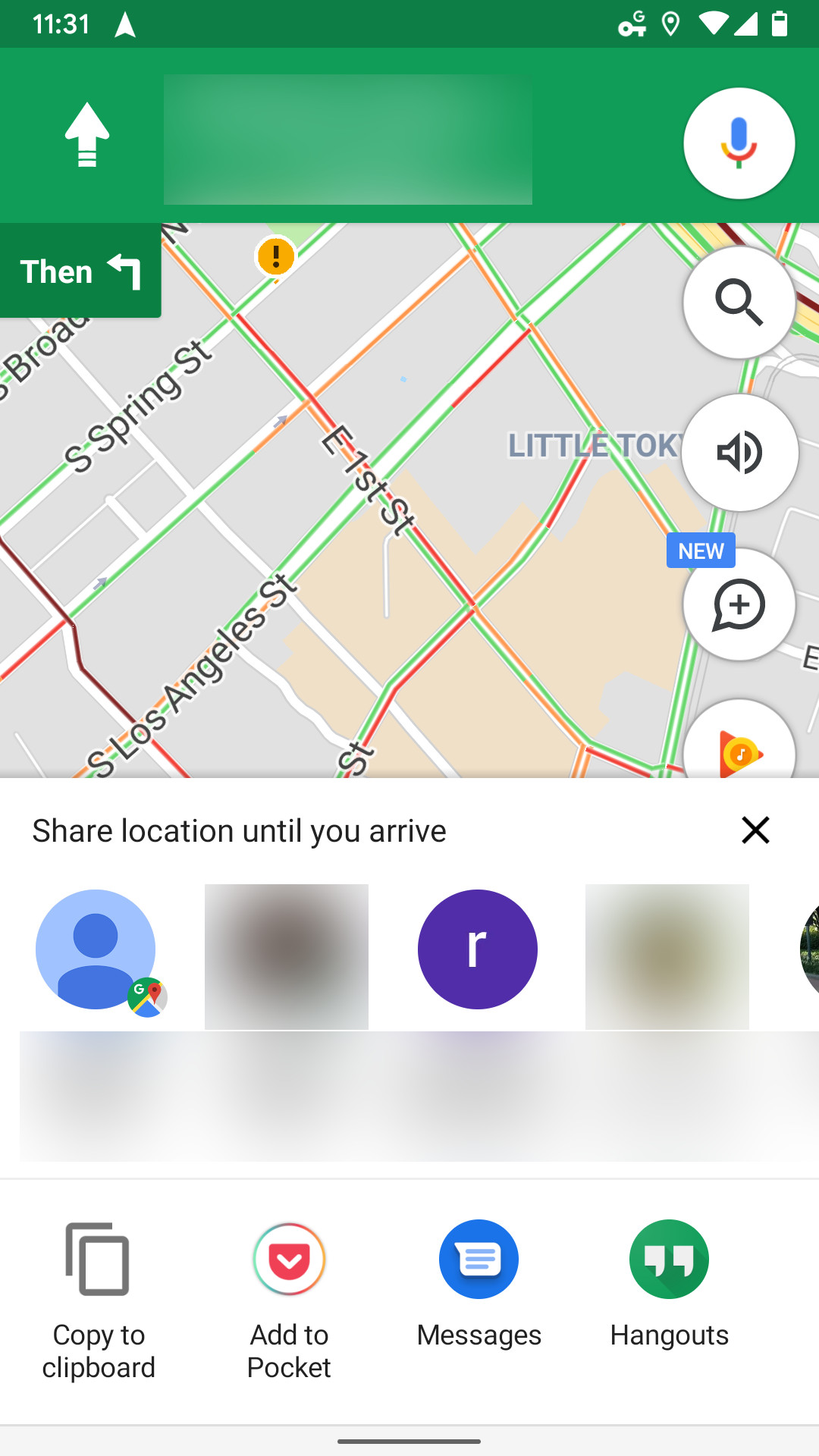This photo, taken with a cell phone, displays a screen that is reminiscent of Google Maps but doesn’t explicitly show the Google Maps interface. In the center of the image, there's a small Google Maps icon subtly placed above the "Share location till you arrive" text. Surrounding this area are profile pictures arranged in a horizontal line, indicating the individuals with whom the user can share their location. Some of the profile pictures are obscured with a blurry square to conceal their identities, and the names of these individuals are similarly redacted with a long blurry rectangle. Below these redactions, four buttons are visible, offering options such as "Copy to clipboard," "Add to Pocket," "Messages," and "Hangouts." The time "11:31" is clearly displayed in the top left corner of the screen.